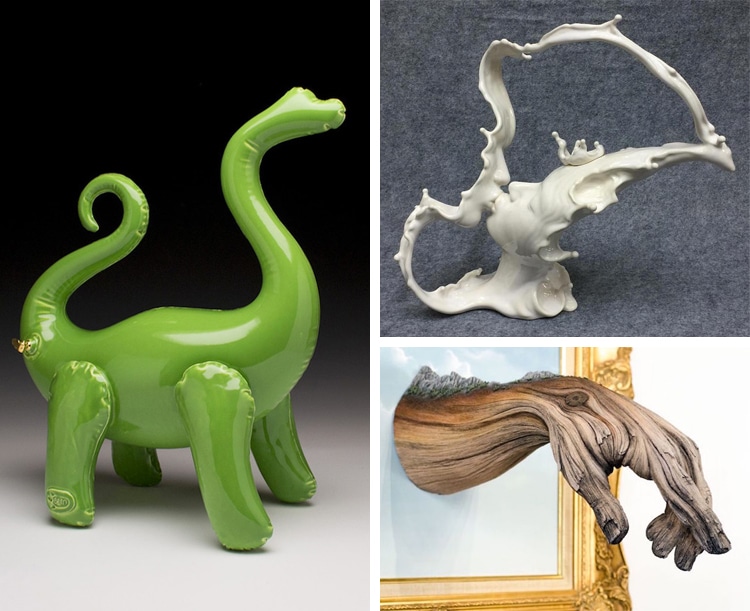The multi-panel image features three distinct sections. On the left side, occupying the largest panel, is a green inflatable dinosaur art piece, characterized by its long neck, curly tail, and visible inflation valve. The dinosaur is set against a black background with a white foreground, looking off to the right. In the top right panel, there is an artistic sculpture of two faces kissing, composed of a white, ceramic-like material that mimics the appearance of spilling liquid, with notable negative space between and around the faces. The bottom right panel showcases a wooden hand, detailed with carved fingernails and gnarled features, emerging three-dimensionally from a golden-framed portrait with a white background, creating a striking visual effect.